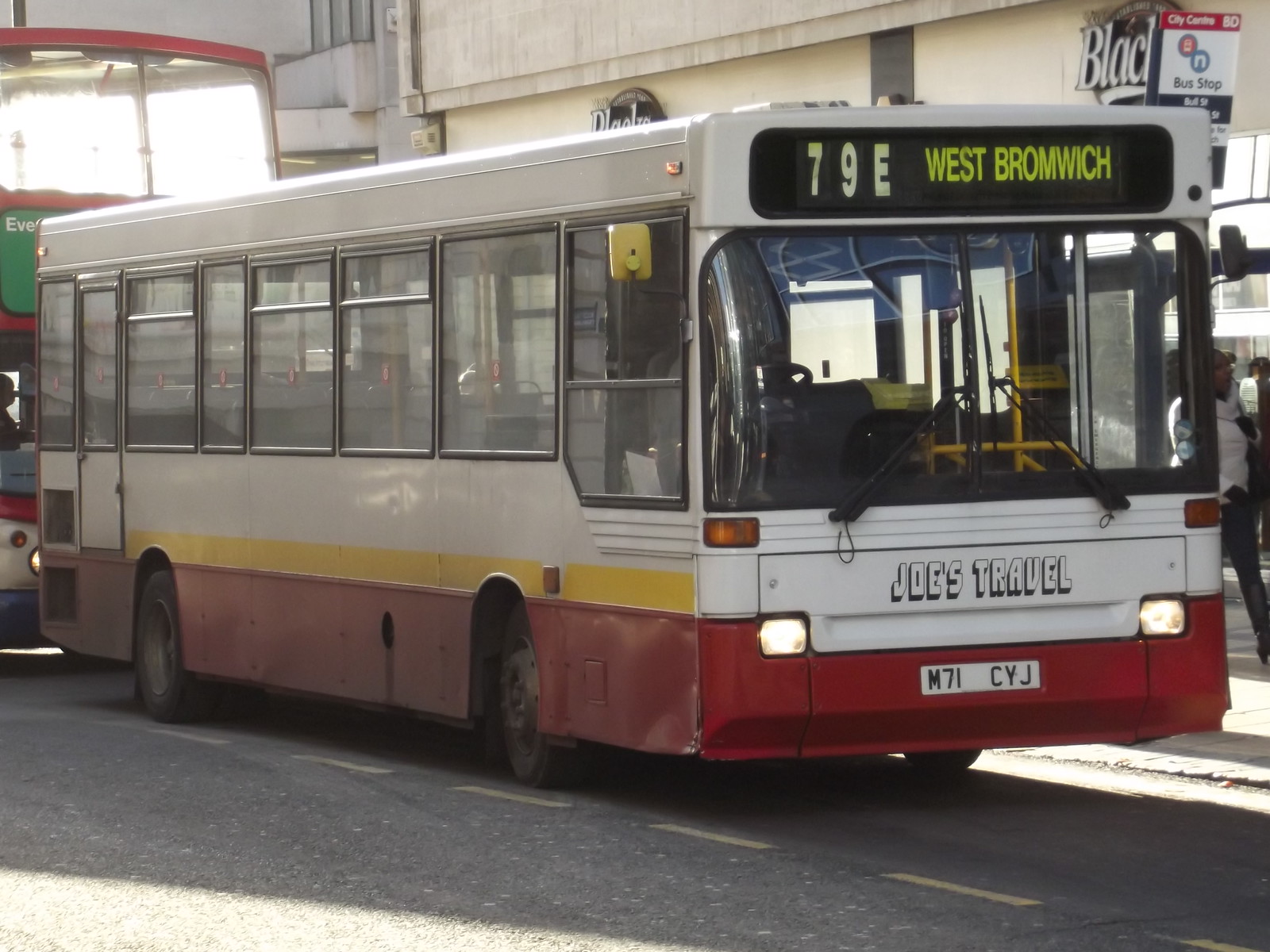The photograph captures a bustling city street scene during daytime, prominently featuring a boxy, somewhat vintage white passenger bus with a bold yellow stripe above the wheels and a red bottom section. Displayed on the front windshield are the words "Joe's Travel" in white letters with black borders, and the license plate M71CYJ is clearly visible beneath. The bus's headlights are switched on. Above the windshield, a digital sign reads "79 East West Bromwich" in white and yellowish-green text. Nearby, a lady dressed in a white turtleneck and black pants stands by the bus. In the background, the front half of a taller double-decker bus, green on top and red around the middle with a white bottom and blue bumper, is partially visible. Surrounding the buses, we can see a stretch of storefronts with noticeable signage, contributing to the urban atmosphere.